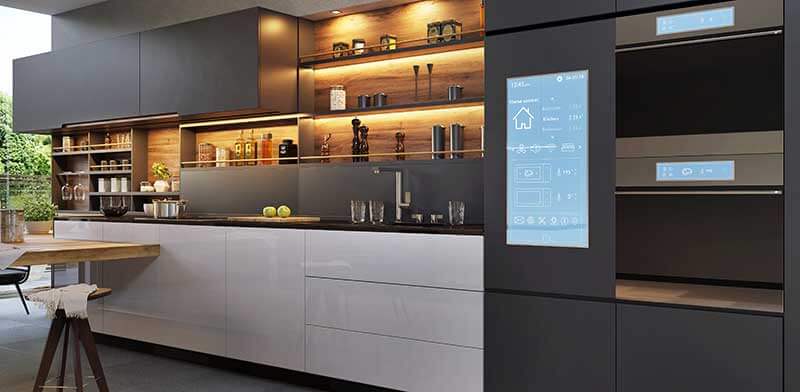This photograph depicts a highly modern and smart kitchen space, characterized by its clean lines and polished look. The kitchen features floor-to-ceiling windows to the far left, revealing a glimpse of green trees outside, enhancing the modern aesthetic. The worktops are a dark black, contrasting sharply with the shiny white, smooth-surfaced cupboards below and the matte dark grey, almost black, overhead units. Shelving is abundant, well-illuminated, and stocked with items like salt shakers. The right side of the kitchen showcases two stainless steel ovens and a high-tech refrigerator with a large touchscreen displaying various controls, indicating an extremely high-tech and programmable appliance. Also noticeable is a digital panel, a mounted touchscreen monitor or computer, a sink, a table, a chair, a stool, glasses, and various light fixtures, reinforcing the overall image of a futuristic, smart home designed for both functionality and style.